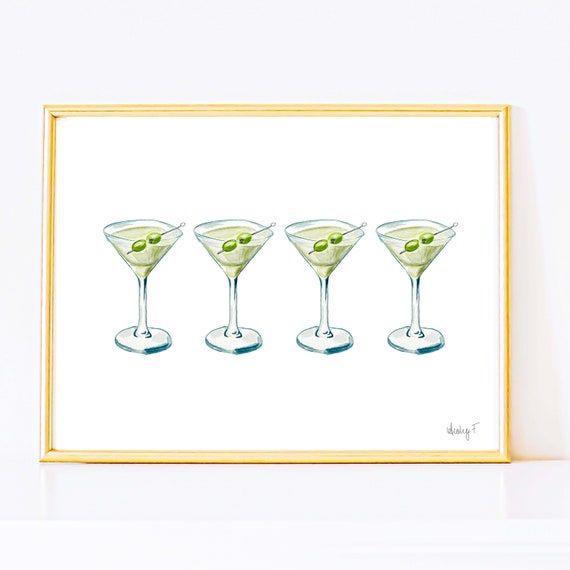The photograph showcases a detailed artwork rendered in line drawing and colored pencils, featuring four identical martini glasses filled with a pale green liquid, likely martinis. Each glass contains a silver skewer accented with two green olives. The background is a crisp white, providing stark contrast to the vibrancy and meticulous details of the glassware. The artwork is enclosed in a metallic gold frame, creating an elegant border that stands out against a light grey background. The artist's signature is delicately placed in the bottom right corner, albeit somewhat small to decipher.